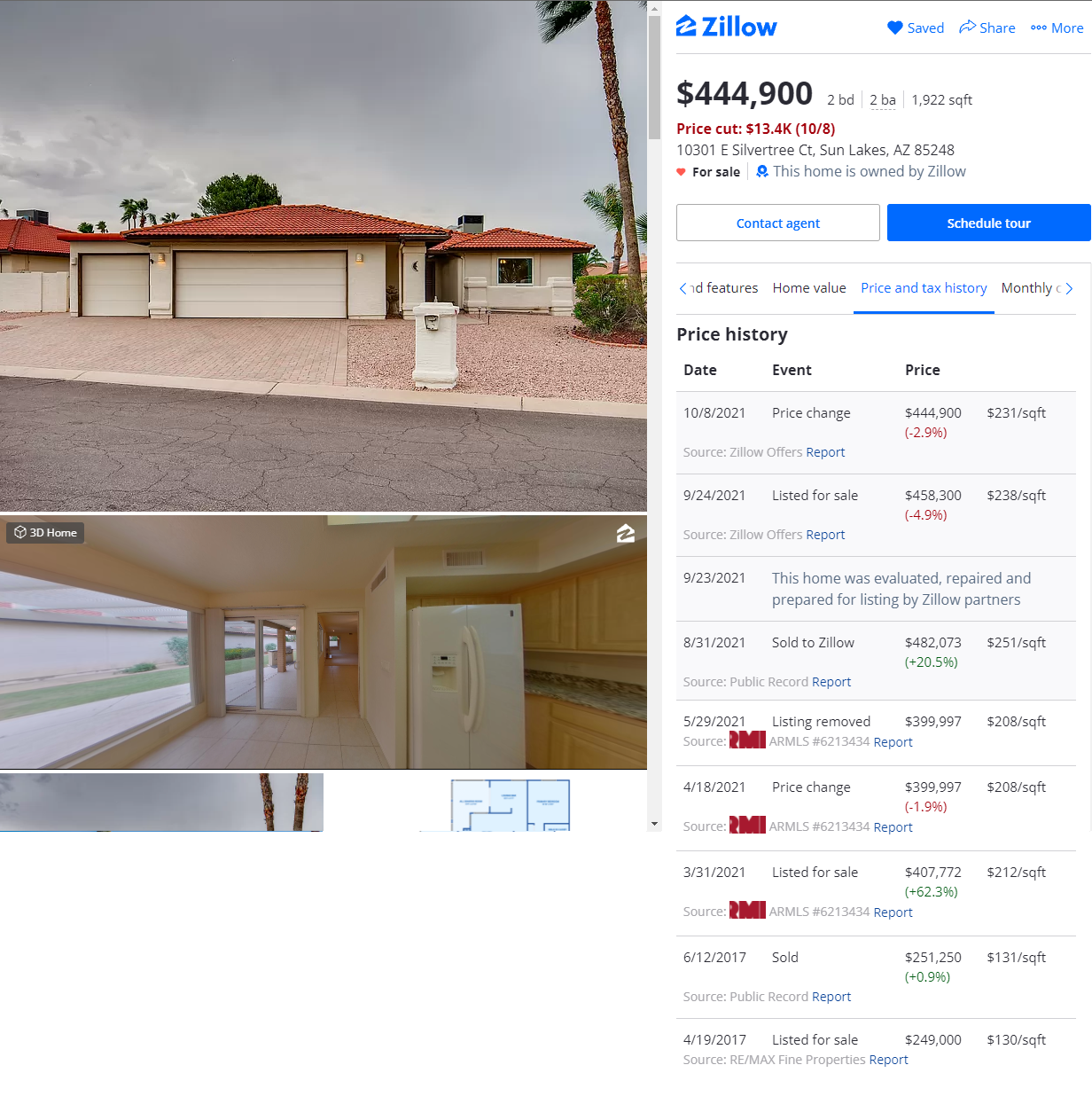In the image, we see a smartphone displaying a Zillow listing. In the upper left-hand corner, there's a prominent photograph of a ranch-style house. The house appears to lack a grass lawn, though the second image in the corner shows hints of green, possibly a small patch of landscaping. To the left, some minimal greenery and a proud palm tree stand against what looks like an overcast sky, hinting at impending rain. The property boasts a unique garage setup with a two-car garage adjacent to a one-car garage.

On the screen, the interior snapshot highlights a spacious kitchen featuring a large picture window. A “3D Home” tag is visible in the corner of this window, indicating that a virtual tour might be available. To the upper right of the screen, the familiar Zillow icon in blue, with a 'Z' inside a house, is displayed prominently along with the 'Saved' tag. Additional options such as 'Share' and 'See More' are available for user interaction.

Scrolling down, the user sees the listing's financial details: the property is listed at $444,900 and comprises two bedrooms and two bathrooms within 1,922 square feet. A note about a recent price cut is visible. Further details include scheduling a tour and extra information, such as historical price data and dates, providing a comprehensive overview for potential buyers.